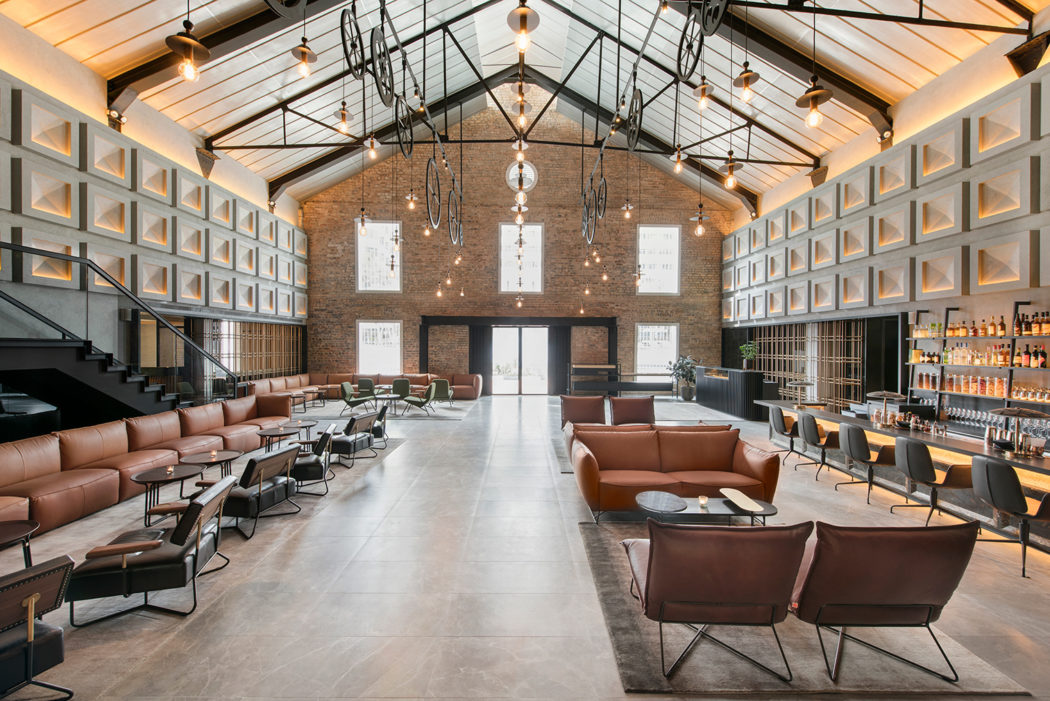The image details the interior of a spacious bar or restaurant with an expansive, high-sloped ceiling reminiscent of an old hangar. The room, comparable in size to a basketball court, features a mix of seating arrangements, including chairs, couches, and padded seats. The left side of the venue contains both leather seating and booth-style seating. A staircase ascending to another room is also situated on the left. The ceiling is adorned with lighting fixtures hanging from structures resembling wagon wheels. Numerous lights hang down from the ceiling, adding to the ambiance. The back wall is constructed of old brick, with three large windows at the top and two sizable windows flanking the double door. On the right-hand side, there is an extended bar area, illuminated from below and stocked with various bottles of alcohol. This bar area includes a closed section towards the back right and an open section at the bottom right. The venue, devoid of any people, appears to be a conceptual or digital sketch, illustrating a potential design for a hotel bar, a restaurant, or a combined coffee shop and bar space.